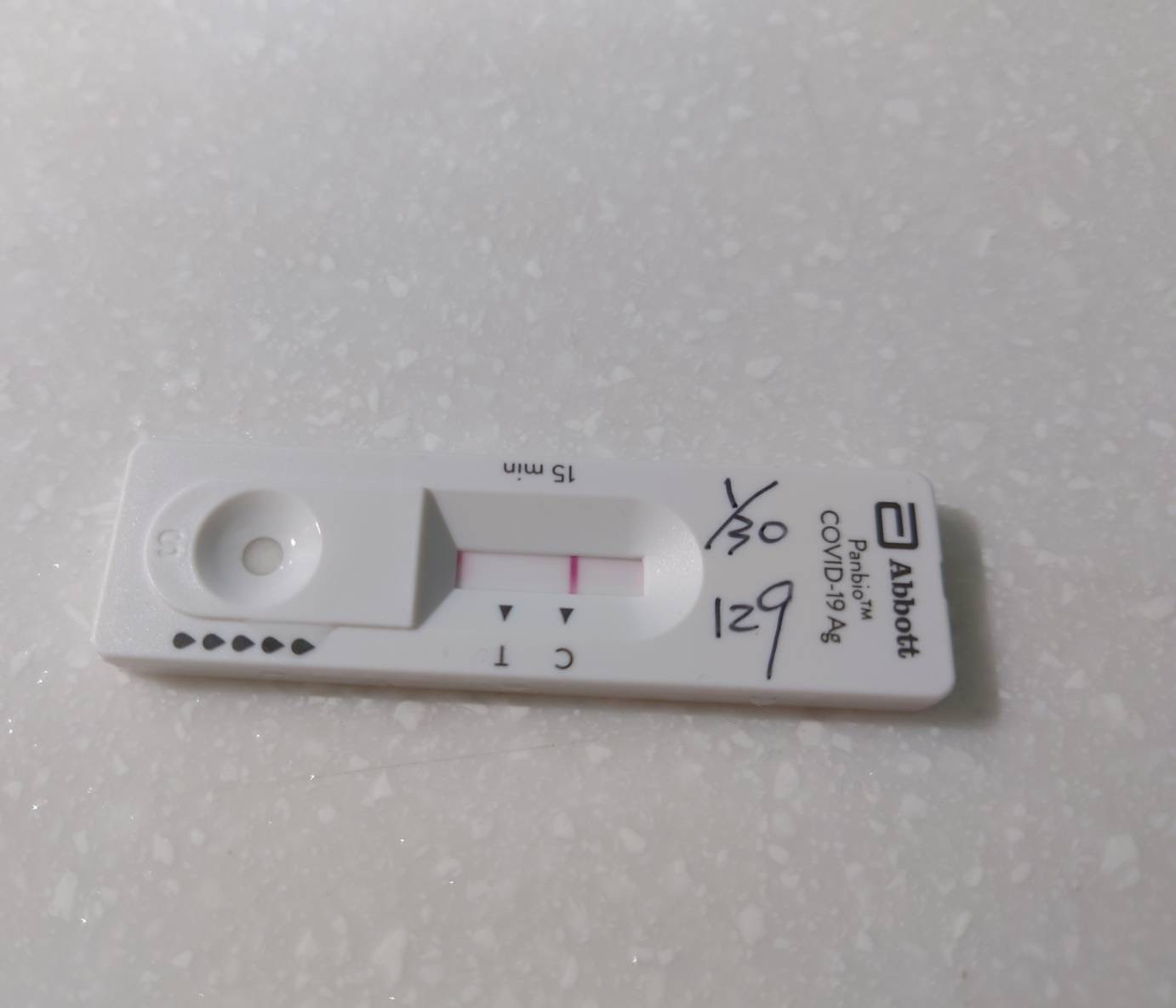The photograph showcases a compact, rectangular COVID-19 test made of white plastic. The surface of the test is marked with various black texts and symbols, providing instructions and designations. Centrally positioned, the recessed test window features a visible pink line labeled "C" (Control) and an adjacent label "T" (Test), which shows no line. To the far left of this window, there is another smaller pink section. 

At the top of the test, the brand name "Abbott" is prominently displayed, followed by the product name "PanBio™" just below it, and then the label "COVID-19 AG." Handwritten in black Sharpie marker, the numbers "1/30" and "129" are clearly printed on the lower section of the test. To the right of the test window, the text "15 Min" indicates the recommended waiting time for the test results.

On the opposite end of the test lies a circular indent embossed with the letter "S" and flanked by five drop-shaped icons, symbolizing the droplet application point. The entire test rests on a textured, white surface, possibly resembling a quartz countertop.